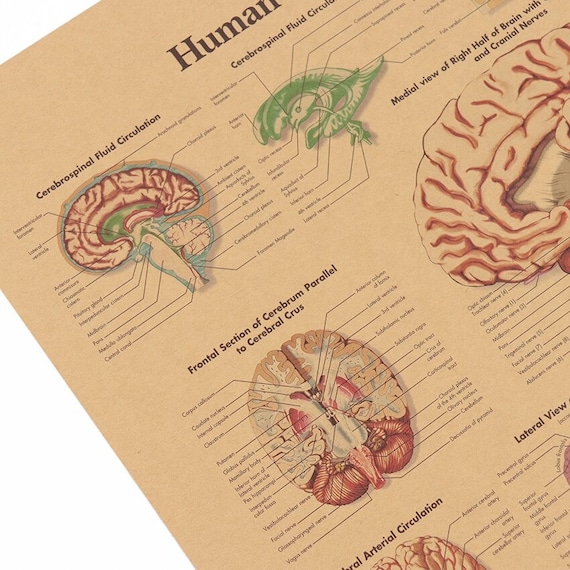This image features a diagonal, tan-colored piece of paper on a white background, depicting various diagrams of the human brain and its anatomy. The top left corner showcases a side-sliced profile view of a brain labeled "Cerebrospinal Fluid Circulation" with black lines and small, illegible labels. Directly below this, there's an overhead view highlighting the frontal section of the brain in red, titled "Frontal Section of Cerebrum Parallel to Cerebral Crust," also annotated with tiny, unreadable text. Further down, part of an image indicating "Arterial Circulation" is visible along with a partially shown and labeled diagram. To the right, another partial diagram labeled "Lateral View" can be seen. Above this, a larger image of brain tissue, prominently labeled "Medial View of Right Half of Brain with Cranial Nerves," takes up most of the space. In the center top of the page, a green diagram again labeled "Cerebrospinal Fluid Circulation" is present. The various parts of the brain diagrams are colored in hues of maroon, salmon, and tan, with some blue tints, all intricately detailed with coordinating lines, though much of the text is too small to be read clearly due to the cut-off sections around the edges of the page.